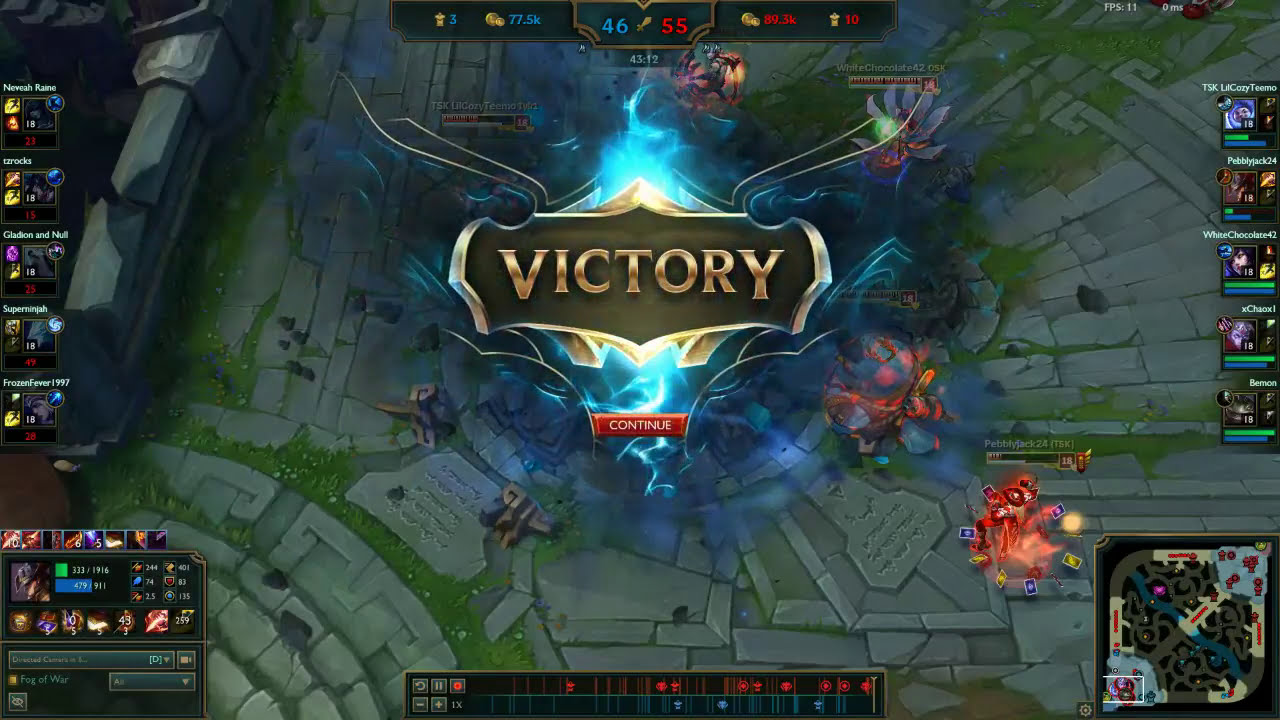The image is a detailed screenshot from a real-time strategy video game, showcasing a victory screen. The elevated camera view captures a courtyard area with an ancient stone surface adorned with intricate decorative patterns, and subtle green moss growing in the cracks. Dominating the center of the screen is a gold-highlighted rectangular box with the word "Victory" in prominent gold text, surrounded by blue flames, and a red button beneath it labeled "Continue" in white text. 

The surrounding interface includes various HUD elements: the bottom right features a map, the right side displays player and team information, the bottom left shows stats, and the top bar displays numbers such as 46-55. The playing field itself has a stone ground interspersed with patches of green grass, along with characters and elements that add a sense of life and interaction to the scene. Some characters on the bottom right are encircled by red flames. This comprehensive ensemble of elements indicates the conclusion of a gameplay session where the blue team emerged victorious over the red team.